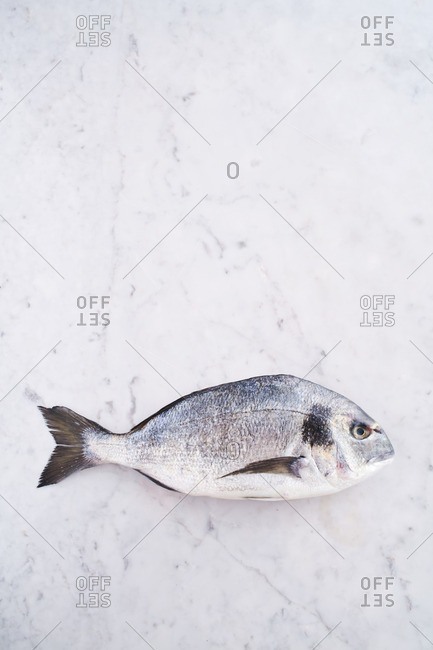This photograph showcases a small, silver fish placed on a white marble surface. The fish, oriented to the right side of the image, features distinctive dark gray fins and tail, a black splotchy spot on its head, and a visibly circular pupil in its eye, which gives it an angry expression. The fish, positioned towards the bottom of the frame, occupies a diamond-shaped section of the marble surface. This section is detailed with text at each corner that reads "offset" in a manner where "set" appears upside down, creating an illusion of "13s." Additionally, one part of the surface displays a plain "zero." The overall color scheme is neutral, dominated by shades of silver, black, gray, and white. The setting hints at possibilities like a meat market, someone preparing to cook, or a store displaying fish.